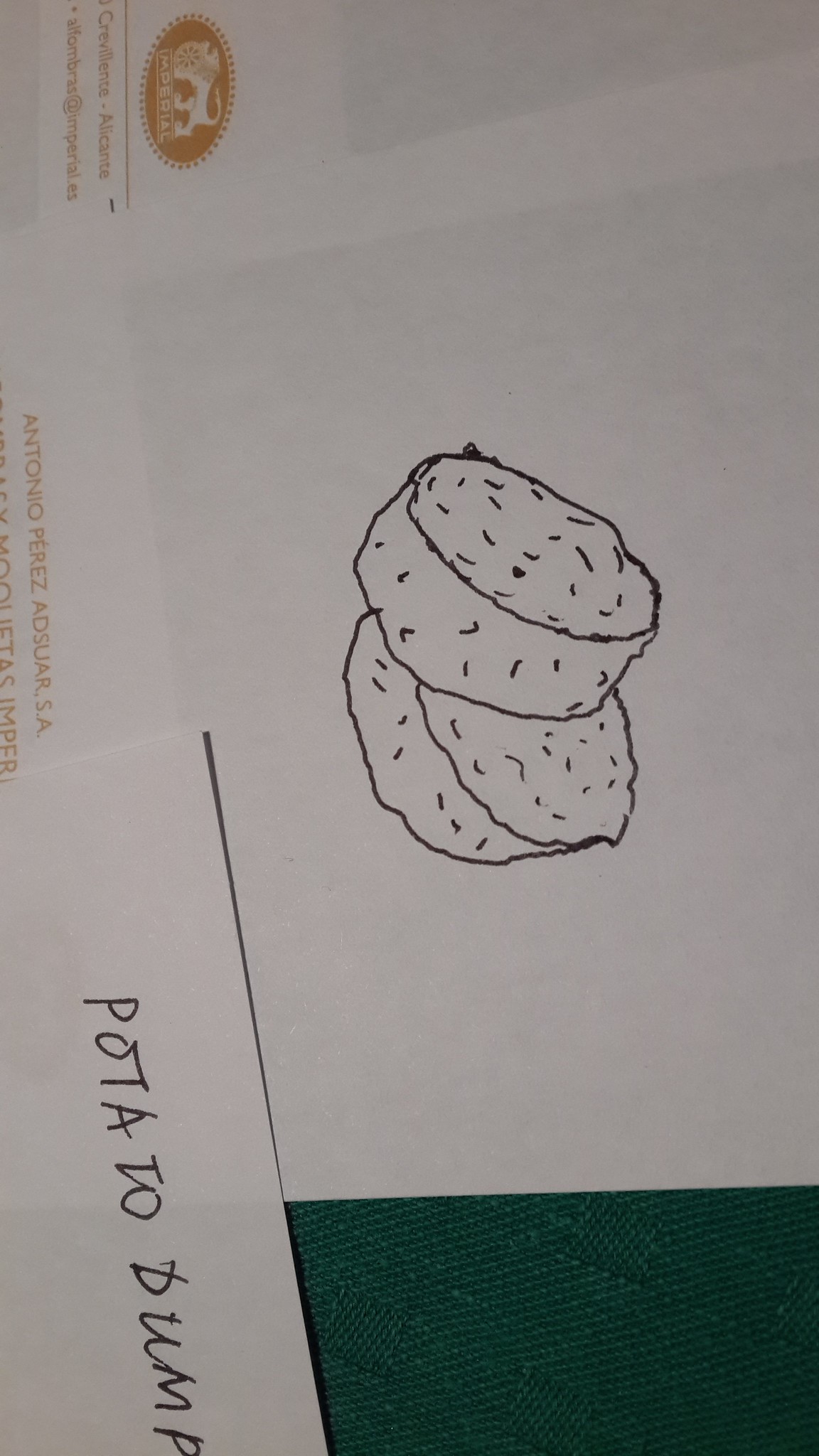This indoor color photograph features a collection of white stationery items arranged on a green surface. Dominating the center, slightly right of the exact middle, is a doodle of what resemble two vertically-oriented biscuits; the biscuit in the background leans to the left, while the one in the foreground leans diagonally, with sides pointing towards the upper left and lower right. The doodle, seemingly created with a black pen, exhibits fine pencil lines detailing the nooks and crannies characteristic of biscuits. Nearby, in the lower right corner, a piece of overlaying paper features the vertically written inscription "POTATO DUMP" in capital letters, also in black pen. The photograph is somewhat dark, but remains sharp, leaving no other words visible except for a letterhead positioned in the lower left corner. This letterhead, vertically oriented, bears the name "ANTONIO PEREZ ADSUAR S.A." in orange lettering. In addition, partially visible is what seems to be another language snippet in burnt orange, which includes an email address: "alfombras@imperial.es."